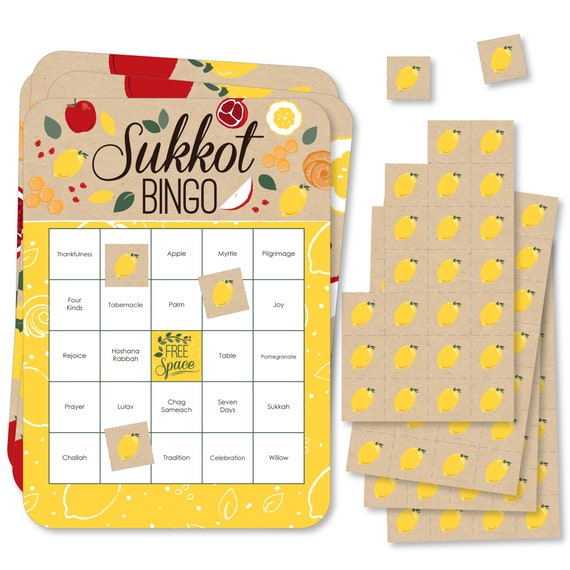The image depicts a close-up photograph of bingo cards against a plain white background. On the left, there are four bingo cards stacked on top of each other. These cards are primarily tan and yellow with a light pink hue, and prominently feature various fruit illustrations including oranges, lemons, and red apples. At the top of each card, in black cursive font, it reads "Sukkot Bingo," followed by "Bingo" in standard font. The layout of the bingo board is visible, with a yellow "free space" in the center. Scattered across the bingo squares are lemon-shaped markers, indicating places where numbers have been called. On the right-hand side, a set of perforated lemon-shaped markers are visible, also stacked and ready for use. Each perforated square is pink with a yellow lemon depicted on it, matching the markers used on the bingo cards. The attention to detail in the fruit illustrations and the stacking of cards and markers create an organized yet vibrant game setup.